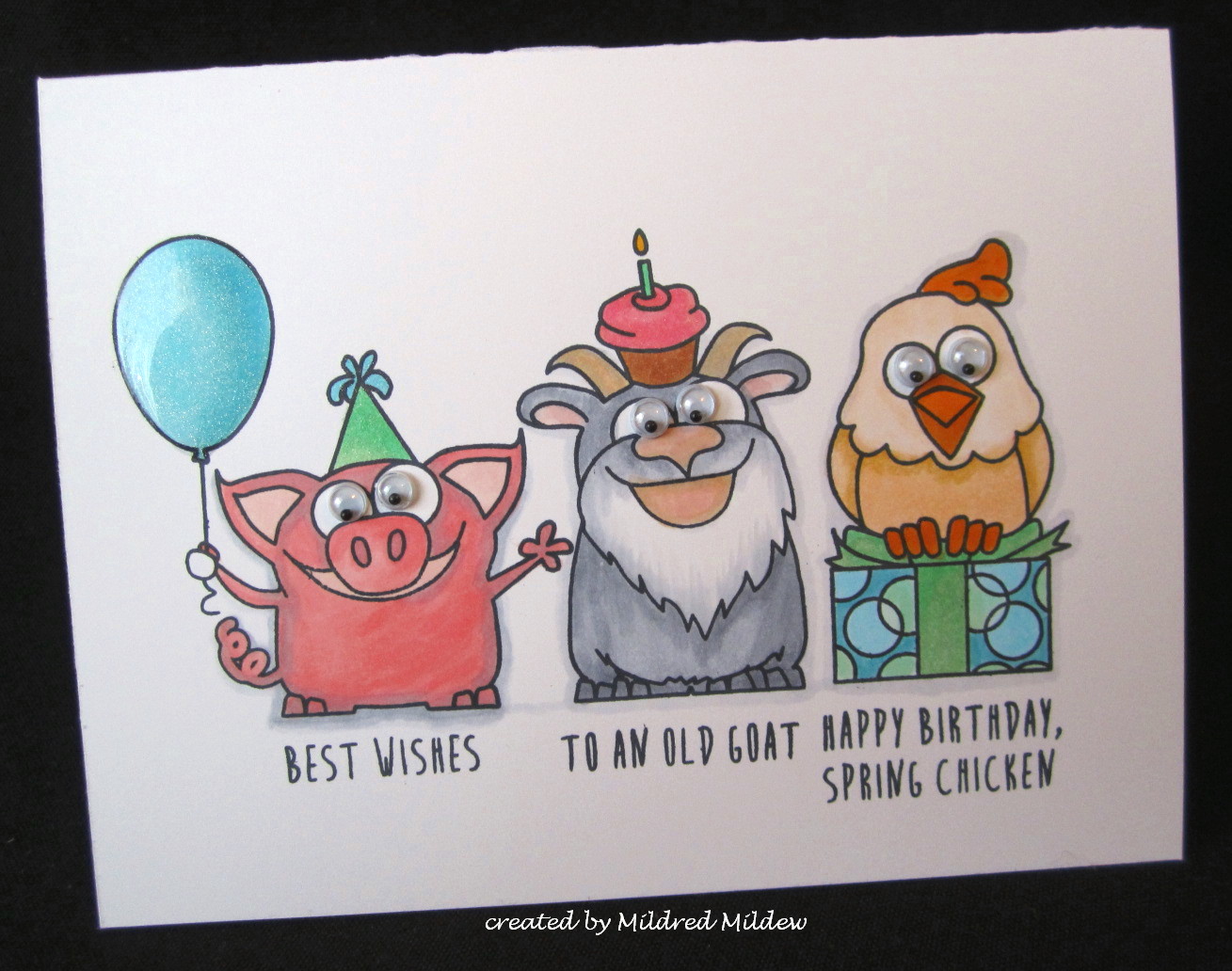This digitally created graphic image resembles a humorous birthday card. It features a black background framing a white center area adorned with animated drawings of animals. On the left, a red pig with pink ears and googly eyes wears a green birthday hat decorated with blue streamers and holds a blue balloon. Below the pig, the text reads "Best Wishes." In the center, a grey, old goat with brown horns, pink ears, and googly eyes balances a cupcake with pink frosting and a lit green candle on its head. The text beneath the goat reads "To an old goat." On the right, a gift box wrapped in green with blue and green circular patterns supports an orange-shaded chicken with googly eyes and red feet. This image is accompanied by the text "Happy Birthday Spring Chicken." Collectively, the text reads "Best Wishes to an old goat, Happy Birthday Spring Chicken." At the bottom of the black border, there's a footnote crediting the creator: "Created by Mildred Mildew."